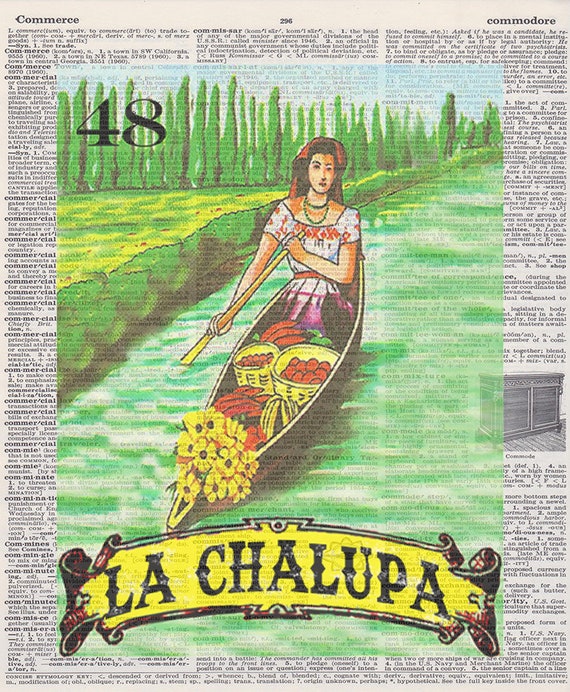This artwork is a detailed painting overlaid on what appears to be a dictionary page in English, with words ranging from "commerce" to "commodore." Dominating the scene is a sketch of a woman in a canoe, paddling alone down a blue-green river. She wears an elaborate dress—white with a red pattern and purple accents—and a headscarf. Around her neck is a green necklace, adding to her colorful attire. She's holding a gold and yellow oar, guiding the canoe which is laden with baskets of produce: red and orange circular fruits or vegetables, yellow fruits or vegetables, and distinctive yellow flowers resembling sunflowers. The lush riverbank features dark green bushes leading to a landscape of yellow and green grass, capped by a line of green trees in the background. The image is bordered by what seems to be a vivid, painted backdrop, and prominently displays the words “La Chalupa” in a fanciful banner at the bottom, with the number 48 in the upper left corner.